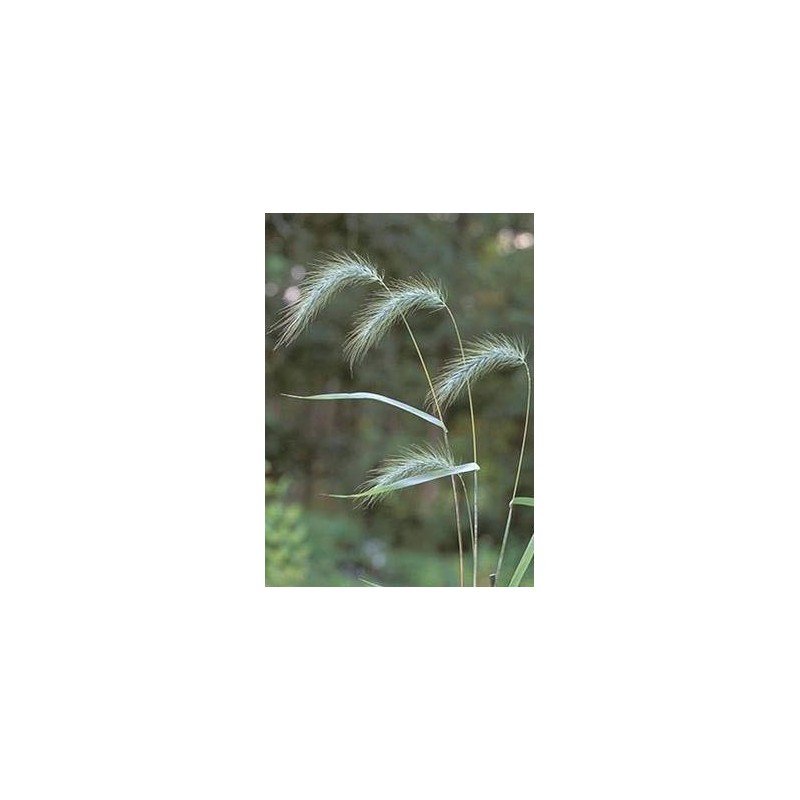This small, vertically rectangular image captures a close-up of a weed, likely Canadian wild rye or a foxtail plant, bathed in natural daylight. The background, composed of blurred, verdant hues suggesting a grassy field with potential trees, emphasizes the prominent weed. The weed itself features very thin yet tall stalks, each topped with a somewhat brown or light green, fuzzy seed formation resembling wheat but curving to the left, possibly due to the wind. Each stalk supports one or two leaves; notably, a thin brown leaf extends from the center towards the left edge, and additional leaves are visible but less pronounced. The intricate details of the plant stand out against the out-of-focus backdrop, creating a sense of movement and natural beauty.